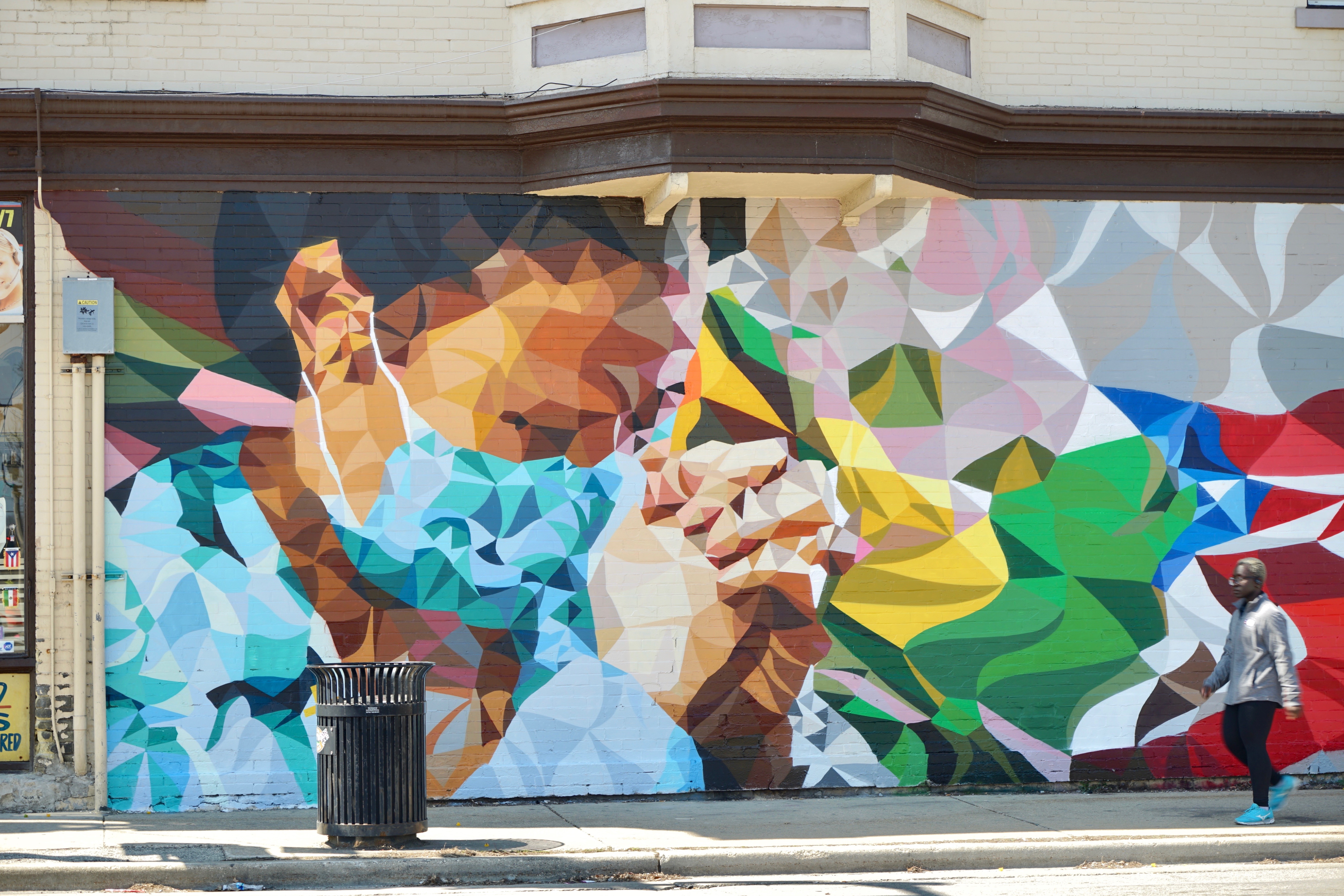The photograph captures a striking mural on the side of a beige building, taken during the daytime. Dominating the mural is a figure with dark skin, black hair, and a blue medical mask and smock, holding their clasped hands close to their face, conveying an emotion of sadness or contemplation. The individual appears to be praying or beseeching. Surrounding this poignant figure are vibrant and varied colors—yellow, purple, green, blues, reds, white, cyan, brown, orange, and black—arranged in a kaleidoscope of geometric patterns including triangles, squares, and squiggly lines.

In the foreground, a man walks along the gray concrete sidewalk in front of the mural. He’s wearing a gray jacket, black pants, and bright teal shoes. His complexion is dark, and he has gray or blonde hair. Nearby, a cylindrical black metal trash bin stands on the sidewalk, and to the side of the mural, beige poles extend upward into a gray fuse box. The overall scene is illuminated by sunlight, emphasizing the lively colors and details of both the mural and the surrounding environment.